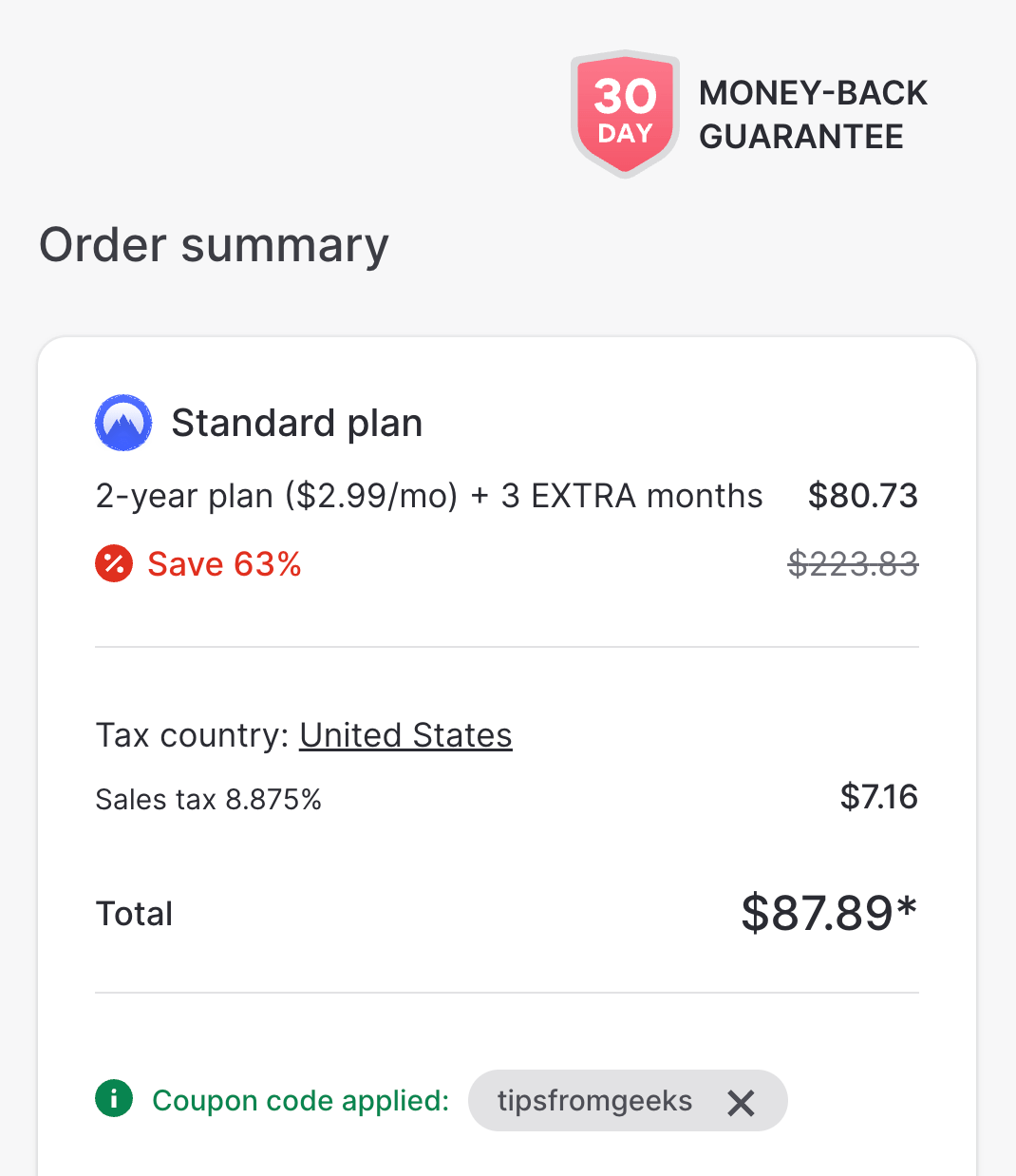A screenshot of an order summary is displayed in the top right corner of the image. The header prominently features a pink shield icon marked with "30 days" in white text, symbolizing a money-back guarantee. To the right of the shield, in bold black text, it reiterates the "money-back guarantee" message. On the left side, at the top, the text reads "Order Summary" in black. 

Below this, there is a large white rectangle that contains the detailed order information. Inside the rectangle, there is a blue NordVPN icon featuring a stylized mountaintop. Adjacent to this icon is the order description in black text, reading: "Standard Plan, Two-year plan, $2.99/month, plus three extra months for $80.73."

To the right of this description, the price "$80.73" is listed in black text. Underneath this amount, the original price "$223.83" is crossed out, and in the same line to the left, there is red text stating "Save 63%."

The next section below lists the tax information. It first specifies "Tax Country: United States," with the text "United States" underlined. Below this, the sales tax rate is detailed as "8.875%" amounting to "$7.16." Following this, the total cost is displayed as "$87.89," marked with an asterisk.

At the bottom of the order summary, in green text, it confirms that a "Coupon code applied," followed by the specific coupon code: "2tips4geeks."